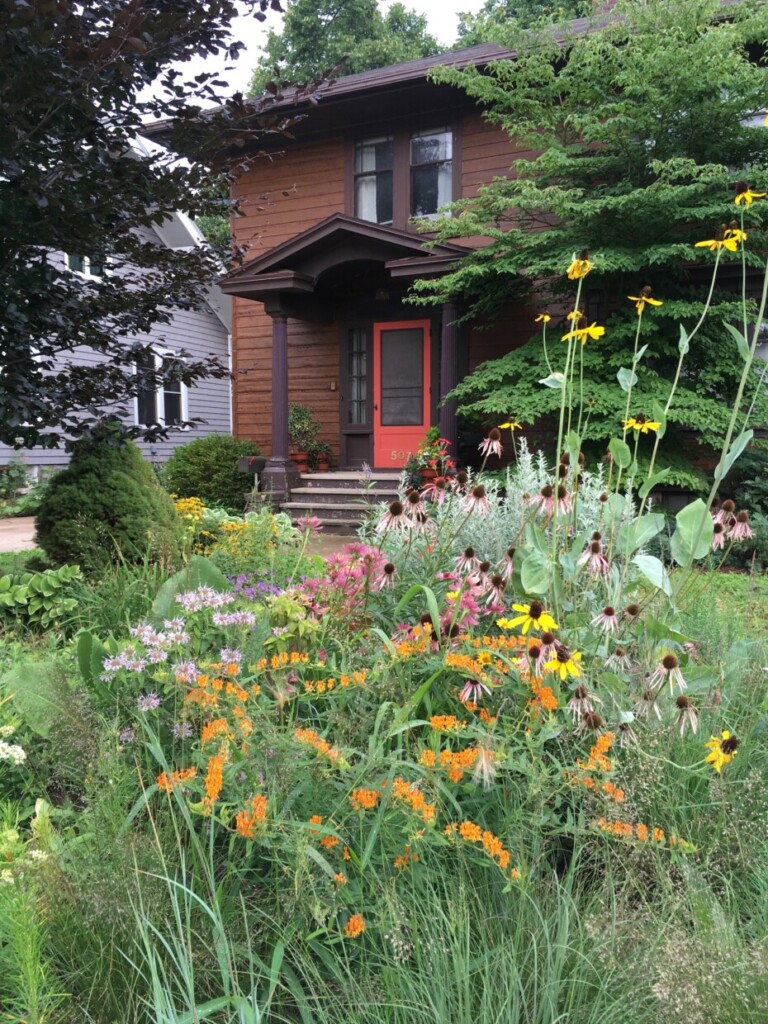The photograph captures the front view of a two-story wooden house with horizontal light brown panels and dark brown trim. The house features a distinct red door and a dark brown patio area with simple columns. Four concrete steps, adorned with potted plants, lead up to the entrance. The yard in front of the house showcases a vibrant, perhaps purposefully overgrown flower garden. This garden is filled with a colorful array of flowers, including sunflowers, orange tiger lilies, black-eyed Susans, yellow daisies, and pink and white blossoms, all interspersed with tall green grass. On both sides of the house, large green trees create a natural frame, with additional trees providing a lush backdrop. To the left of the house is an adjacent gray, possibly dusty blue, building with a white roof and windows. The photograph, taken in daylight under a cloudy sky, vividly portrays the lively and well-maintained exterior space.